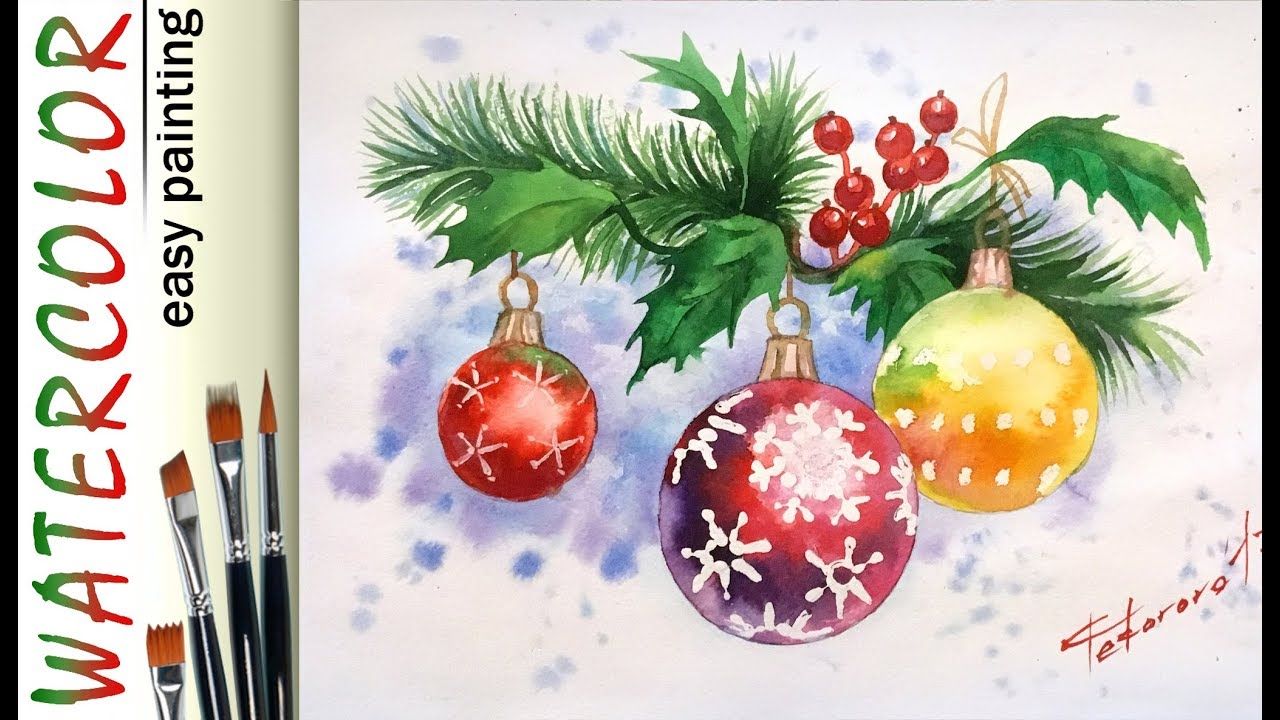This image depicts the cover of a book titled "Watercolor Easy Painting," with the words "watercolor" in red and green text and "easy painting" in black text. The illustration on the cover features three Christmas ornaments hanging from a branch. The ornaments consist of two red ones and one gold one, each decorated with white designs; the red ornaments showcase snowflakes, and the gold ornament is adorned with polka dots. These ornaments are depicted hanging from sprigs of mistletoe, complete with red holly berries. Additionally, four clean paintbrushes are neatly arranged at the bottom of the image's left side. A signature is visible in red in the bottom right corner of the artwork, adding a personal touch to the festive scene. The background is predominantly white, with hints of blue that add depth to the composition.